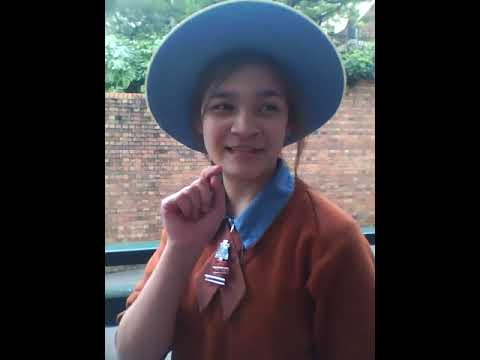This photograph captures an outdoor scene where two young girls, likely schoolmates, are seen sitting and laughing on a bench. Both girls are dressed in similar school uniforms consisting of maroon long-sleeve sweaters over blue collared dresses, with the dresses appearing to fall below the knee. The girl on the left is wearing black shoes with white ankle socks and a blue hat. Her glasses complement her bright, laughing expression. The girl beside her, seated on top of the table portion of the bench, is also smiling warmly, though only the lower part of her face is visible. The bench is cluttered with various items, including school books, glasses cases, and a cell phone. In the blurry background, other individuals wearing identical uniforms suggest a school setting, adding to the lively and joyful atmosphere of the image.